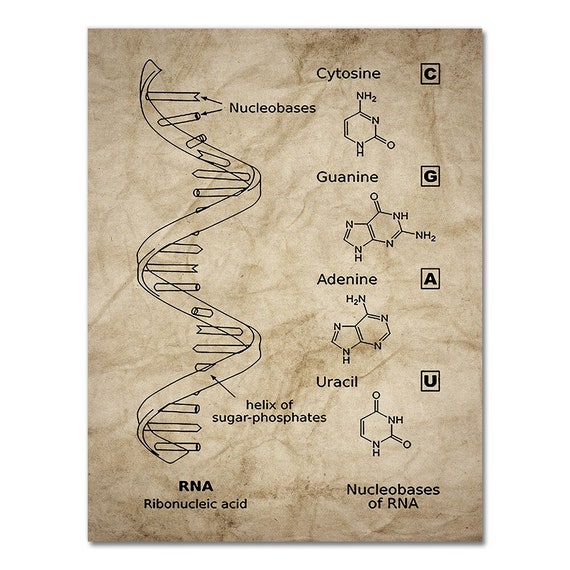The image is an aged, yellowish-brown sheet of paper featuring a detailed scientific diagram related to RNA (ribonucleic acid). The central focus is on the single helix of sugar phosphates which is illustrated on the left side of the image, resembling a spiral staircase with arrows pointing to various components. The diagram includes detailed labels and arrows pointing to the nucleobases: Cytosine (C), Guanine (G), Adenine (A), and Uracil (U). Each nucleobase is depicted with its chemical structure, including labels like NH2, N, and O in different corners of the hexagonal shapes. Cytosine is shown within a square, Guanine has two interconnected hexagons, Adenine also has two hexagons, and Uracil is represented with a single hexagon. To the bottom left of the image, the text "RNA" is written, with "ribonucleic acid" in smaller font below it. The right side of the diagram is dedicated to illustrating how these nucleobases are part of the RNA structure, emphasizing their scientific makeup and how they fit together in the RNA strand.